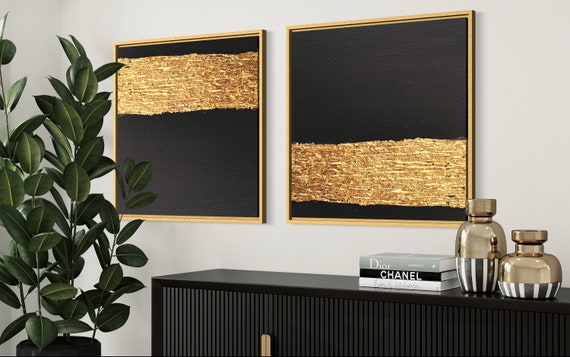The photograph showcases a living room with light grey walls adorned by two square pieces of artwork in gold frames. The artwork is predominantly black, featuring a notable gold band—one piece has the gold stripe across the top half while the other features the stripe near the bottom. To the left of the artwork is a tall green plant, adding a natural touch to the room. Below the paintings, a wooden stand with striped patterns and a handle serves as a focal point. On the stand, there is a neatly arranged stack of three books: one labeled "Dior," another "Chanel," and an indistinguishable third book. Accompanying the books are two jars, characterized by their goldish hue and grey and white vertical stripes.